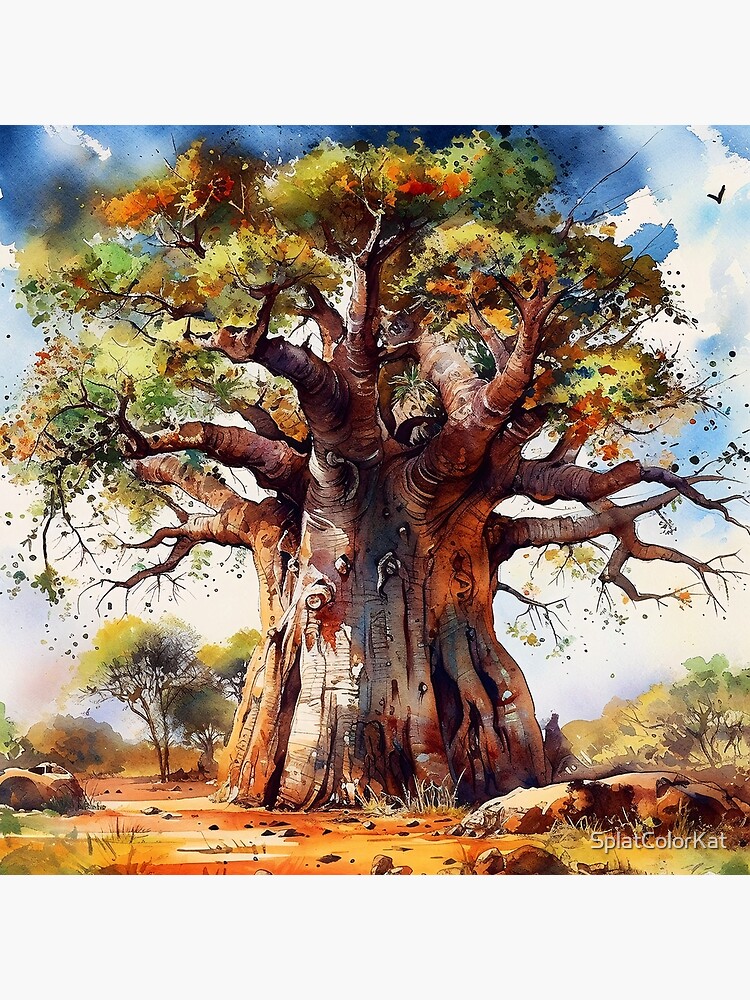This watercolor illustration features a massive, ancient-looking tree that resembles the iconic Baobab tree or the Tree of Life at Disney World. The trunk is exceptionally wide and thick, splitting into equally robust branches that spread out to create a dense canopy. The tree is not very tall but is particularly remarkable due to its immense girth. The foliage at the top consists of a mix of light green, orange, yellow, and some red leaves, giving the tree a vibrant, multi-hued appearance.

The background sky is a clear blue, dotted with white clouds, and a small black bird can be seen flying to the top right of the tree. The ground beneath the tree is covered with scattered rocks and has an orangish soil. Surrounding the central tree are thinner trees with greenish, yellowish, and brownish leaves. At the bottom right corner of the illustration, there is a watermark stating "Splat Color Cat."